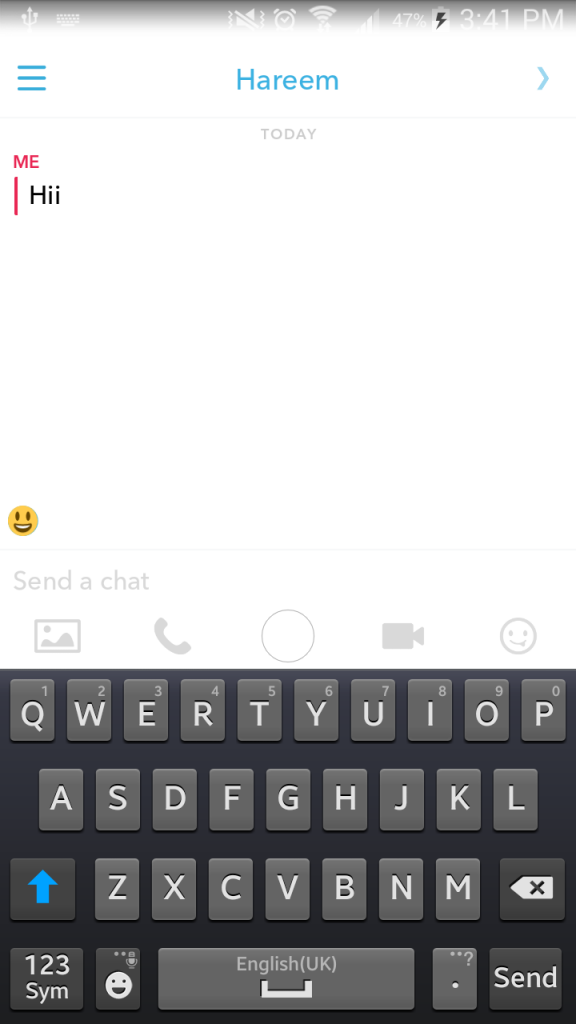The image depicts a smartphone interface set in portrait mode, showcasing a messaging application. At the top left corner, there is a small keyboard icon, indicating that the keyboard is active. On the right side, a series of status icons are visible: an alarm clock, a muted sound icon, Wi-Fi and reception signals, and a battery icon displaying 47% with a black lightning bolt, suggesting the phone is charging. The current time, 3:41 PM, is also shown.

Beneath the status bar, the app interface displays a profile named "Harim" in blue text on the left, accompanied by three blue lines. To the right of the name, there's a blue arrow pointing to the right. Below this header, the word "Today" appears, followed by a chat message displayed in red text labeled "me" and containing the message "hi" with two eyes in black text.

At the bottom of the chat window, there is a smiley face icon and the phrase "Send a chat" in gray text. Several symbols are also present: a picture icon, a phone icon within a white circle, a gray camera icon, and a smiley face icon. The active keyboard is gray with a QWERTY layout, featuring a blue arrow button pointing up and the spacebar labeled "English UK." To the bottom right of the keyboard, the send button is visible.